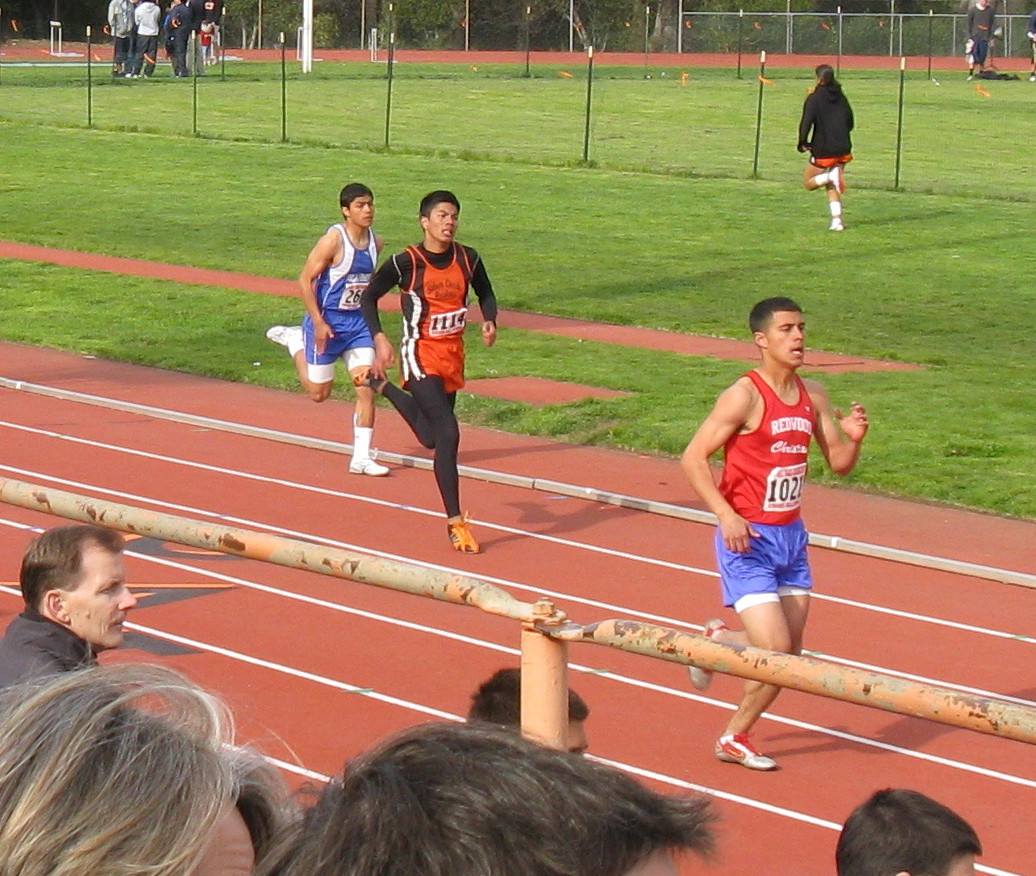This is a photograph of a lively track and field event featuring three men racing on a straight section of the typical red clay track. The grassy center field, enclosed by a weathered iron fence, adds a splash of green to the scene. Spectators, their attention riveted towards the right, perhaps where the finish line lies, are visible on the opposite side of the fence with the tops of their heads peeking into view.

In the race, the leading runner sports a red tank top and light blue shorts, numbered 1021, mid-stride with short black hair. The second runner, grimacing with intense focus, wears a unique combination of an orange tank top over a long-sleeved black top and black leggings, paired with orange shorts and marked with the number 1114. The final runner, the third in line, dons a blue tank top and blue shorts with white socks, characterized by short black hair and a determined posture with one leg raised high.

In the backdrop, the track loops around to the left, melding into the distant tree line, while a few people casually linger on the grassy field in the center. This colorful scene captures the essence of intense athletic competition, communal support, and the rustic charm of the track facilities.